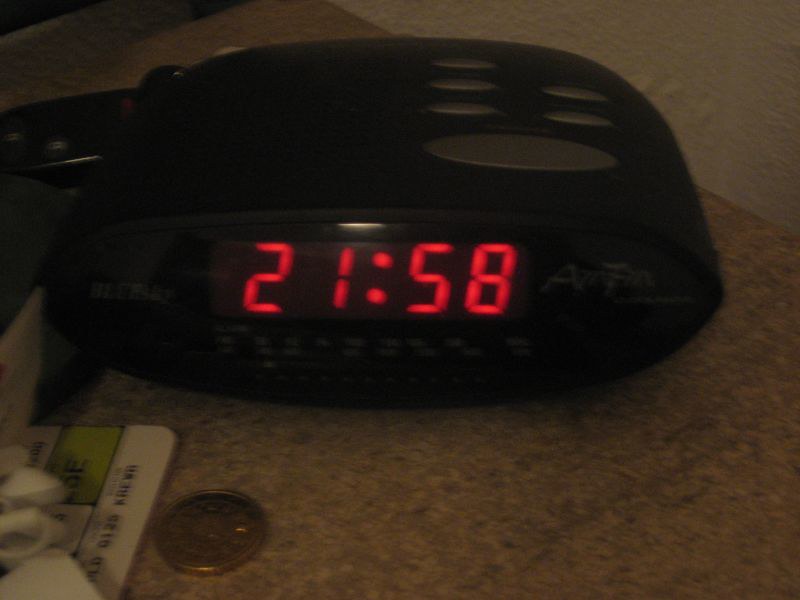This real-life photograph captures a digital clock positioned on what appears to be a granite surface, viewed from an angle that showcases both the top and front of the device. The clock has an oval shape and is predominantly black in color. Prominently featured on the top are several silver oval buttons: one large button at the forefront, followed by a column of three smaller buttons and an adjacent column of two smaller buttons.

On the clock’s display, the time "21:58" is vividly presented in red digits against a black digital screen. Adjacent to the display, there is faint white text reading "AM FM," although additional smaller text is not legible due to the image's graininess. Below the time display, there is an indication of a radio station dial, though specific numbers are indistinct and faded.

The clock rests on a granular surface resembling granite, surrounded by a few items including a copper-colored coin, similar in size to a quarter, and partially visible pieces of paper. The photograph's graininess obscures some details, making it challenging to decipher smaller text and elements around the clock.